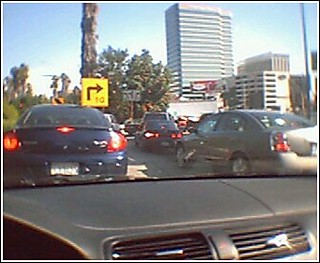A vintage photograph taken from the driver's seat of a car captures a bustling urban scene. The image features a line of vehicles waiting to either make a right-hand turn or merge onto a new route. The dashboard of the car, visible at the bottom of the frame, suggests the photo dates back to an older era. In front of the driver, a variety of cars, including a large semi-truck in the background, are queued up with their brake lights illuminated. The surrounding cityscape is characterized by tall buildings and intermixed with trees, painting a picture of an urban environment. A prominent yellow traffic sign warns of an upcoming right-hand turn, contributing further to the authenticity and context of the image.